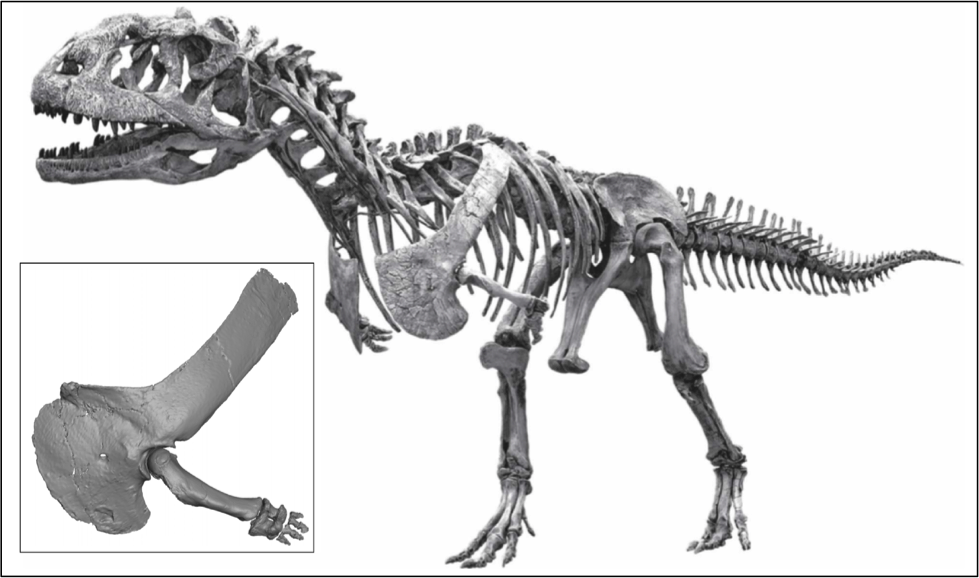The image presents a detailed skeleton of a dinosaur, identified as an Allosaurus, displayed against a stark white background. The skeleton is meticulously arranged to showcase the dinosaur's anatomy, with its head featuring prominently in the top left corner of the horizontal rectangle. The open-mouthed head points leftward, while the long tail swoops down slightly and extends to the right edge of the image. The Allosaurus is positioned centrally and is depicted standing on its two robust legs, further highlighting its formidable stature.

An inset, a small square outlined in black, is situated in the bottom left-hand corner of the image. This inset zooms in on the dinosaur's tiny hands, providing a close-up view of the intricate structure of the short arm and its attached bones. The entire fossil structure and the inset share a gray coloration, emphasizing their stone-like preservation. The thin gray line outlining the overall image, coupled with the white background, accentuates the fossil, making it the focal point. The visual presentation, enriched by these details, serves as a compelling depiction of extinct animals, emphasizing the distinctive features of the Allosaurus skeleton.